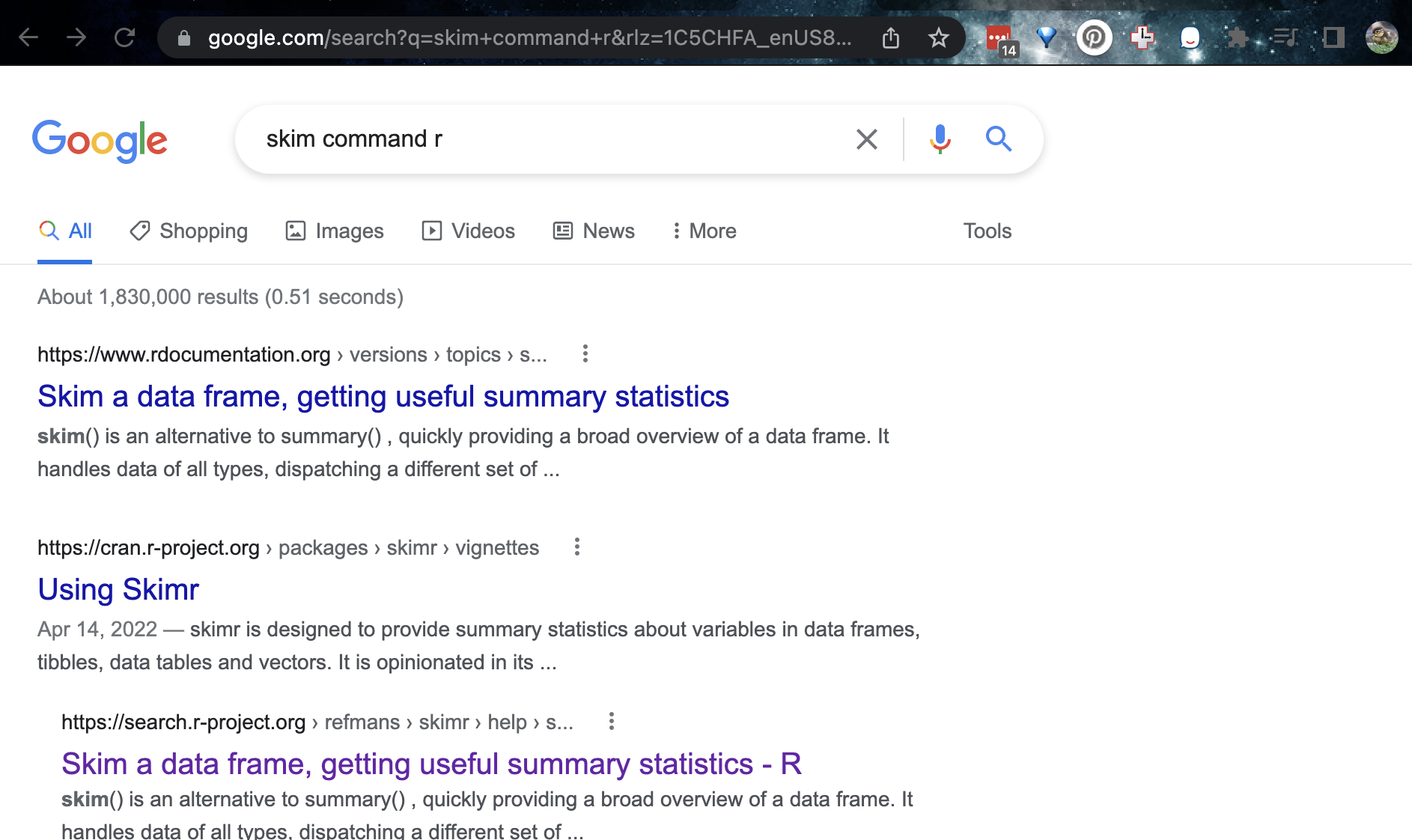The image features a user interface that appears to be a search engine results page. At the very top, there is a black rectangle serving as a header or toolbar. On the left-hand side of this header, an arrow points left and another points right, along with most of a circle featuring an arrow at its end, suggesting navigation tools. Nearby, there is an icon resembling a lock followed by words and a symbol that are not clearly identifiable. A star icon is also visible.

The background of the page is primarily blue and white. There is a red square with a gray square overlaid on it, featuring several small dots. Additionally, there's a notable blue shape on the page. A white circle with black content inside it is present, along with an object that resembles a cross with hands similar to a clock. Another white circle contains what looks like a red dot.

Several gray symbols are scattered around, though they are not easily discernible. There’s also another circle with some intermediate details within it.

On the left-hand side, the word "Google" is displayed in its characteristic multi-colored font. A gray-outlined rectangle that bulges at the sides includes written text and an "X" on the right-hand side, presumably for closing the rectangle. This section also contains a microphone icon and a magnifying glass, the latter indicating the search function. Beneath this, there’s another magnifying glass icon followed by the word "All" highlighted in blue with an underline.

The page displays navigational tags such as "Shopping" adjacent to a tag icon, "Images" next to a square with an image symbol, "Videos" besides a square with an arrow, "News" represented by a square with lines in it, and "More" symbolized by three vertically aligned dots. There is also a label for "Tools".

Below these navigational elements, search results begin to appear. The first result has the title "Skim a Data Frame: Getting Useful Summary Statistics" in blue text, with accompanying descriptive words beneath it. Following this is another result, featuring "Using SKIMR" in blue text, surrounded by additional text. There are also clickable website links in purple, with related descriptive text underneath. The visible text in one of these excerpts includes "Skim a Data Frame: Getting Useful Summary Statistics - R."

Interspersed throughout the results, there are several instances of three vertically aligned dots, indicating more options or settings related to individual search results.